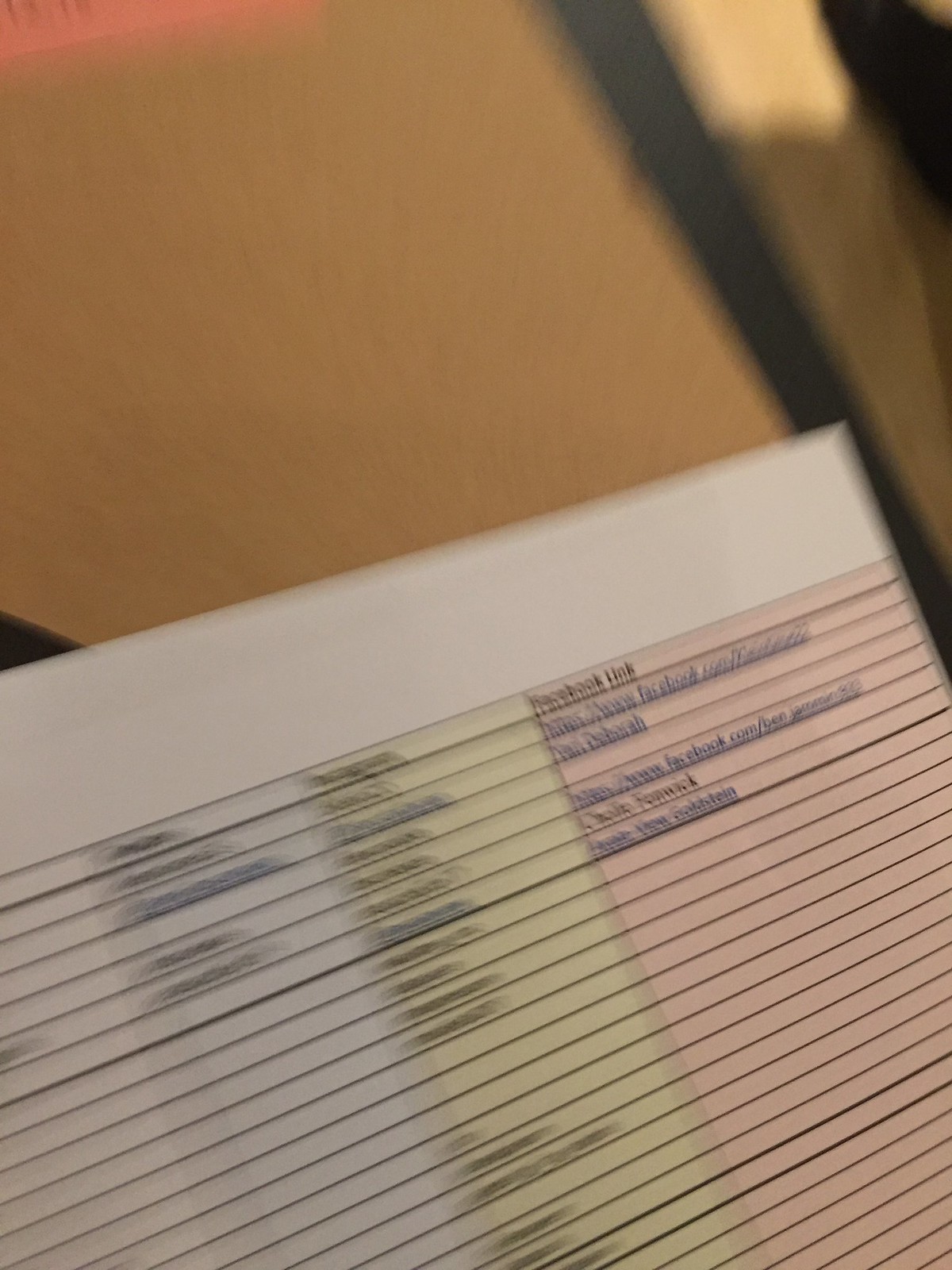The photo depicts a blurry printout of a document on what appears to be a tan desk or possibly an area with a brown background, such as a bulletin board. The document is organized into four vertical columns of different colors. The first column on the left is white and has some illegible text, followed by a light blue column containing four or five labels. The third column is yellow, featuring about 13 to 14 items, though the text is not clear. The fourth column on the far right is pink, twice as wide as the other columns, and includes five or six items. Notably, this column houses a header that seems to mention a "Facebook link," partially visible with an "HTTPS" web address format. The document resembles a table or spreadsheet, with horizontal and vertical lines segmenting the various entries within each colored column. Overall, the image's blurriness severely limits readable details, but the colored sections and the partial text offer some insight into the document's structured layout.